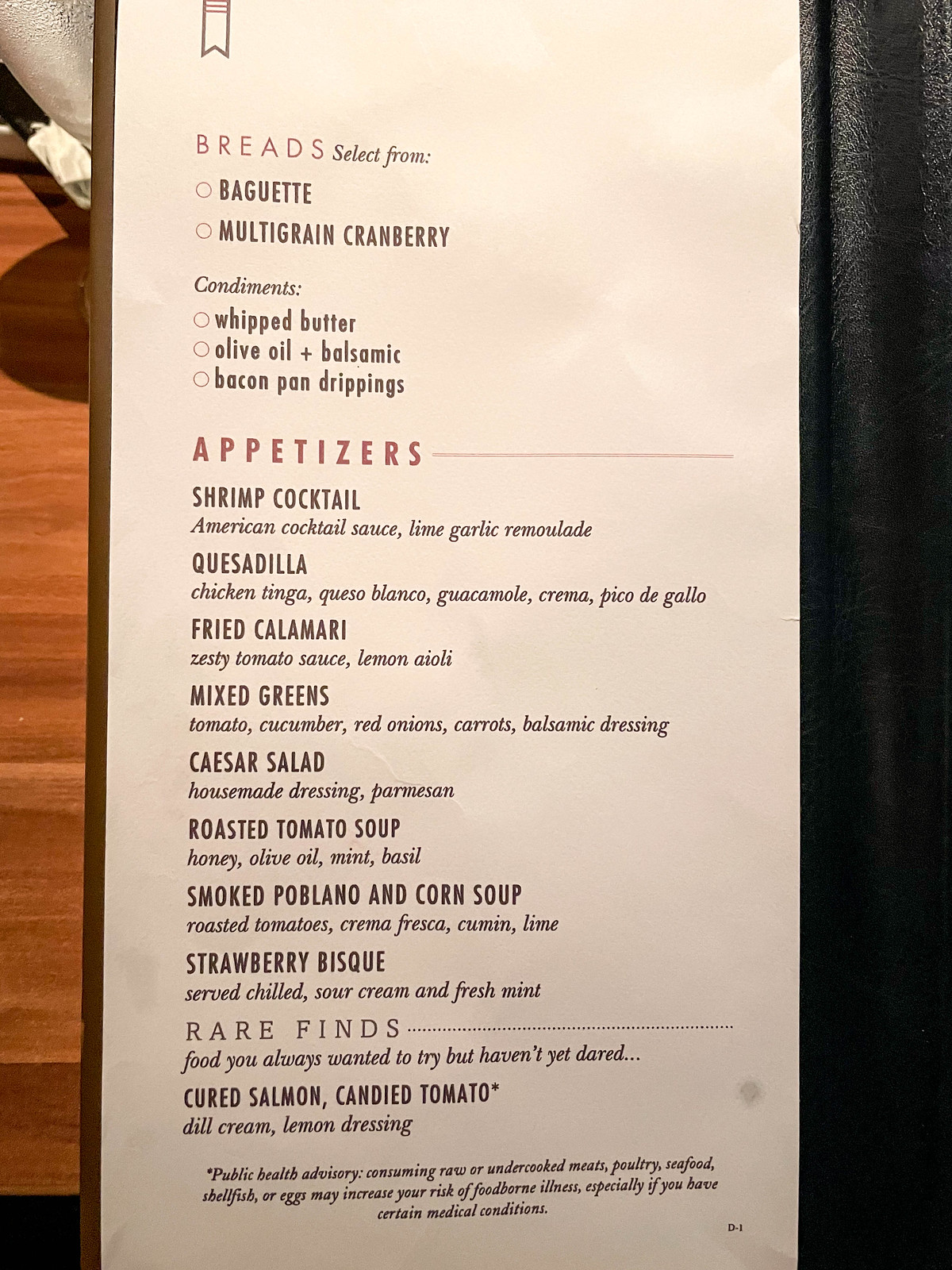This photograph captures a restaurant menu displayed upright at the edge of a wooden table. The menu is held within a sleek black plastic cover, and a delicate ribbon adorns its top left corner, adding a touch of elegance. The menu itself is a clean white with predominantly black text, complemented by touches of red and white for emphasis.

At the top of the menu, under the heading "Breads," diners are invited to choose between a "Baguette" and "Multigrain Cranberry." Below this, the "Condiments" section offers "Whipped Butter," "Olive Oil plus Balsamic," and "Baked Pan Drippings."

Highlighted in a light red hue, the "Appetizers" section features a variety of starters: "Shrimp Cocktail," "Quesadilla," "Fried Calamari," "Mixed Greens," "Caesar Salad," "Roasted Tomato Soup," "Smoked Poblano and Corn Soup," and "Strawberry Bisque."

Following this, under the section titled "Rare Finds..." with an ellipsis for dramatic effect, the menu lists gourmet items such as "Cured Salmon," "Candied Tomato" (marked with an asterisk), "Dill Cream," and "Lemon Dressing." At the bottom of the menu, an asterisk leads to a public health advisory, informing customers of potential allergens or health considerations.

In the background, the rich texture of the wooden table adds warmth to the setting, enhancing the overall dining ambiance captured in this photograph.